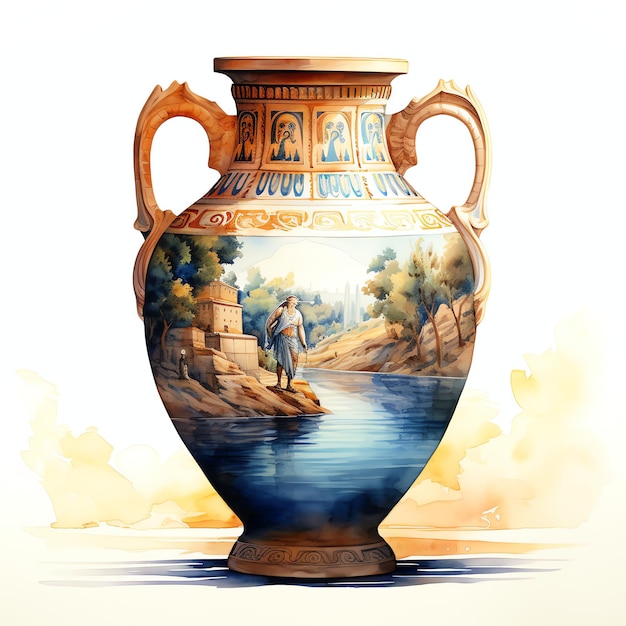This is an intricately designed Grecian-style vase, likely a watercolor painting or illustration. The vase has a traditional shape with two handles near the top, tapering down to a narrow base. A round center broadens towards the middle before tapering, giving it a jug-like appearance. The handles and top are beige with darker brown hues featuring a repeating border pattern of stylized images, possibly faces and teardrops. The overarching background of the vase transitions from a white top to a yellowish hue towards the bottom, with a blue shadow or watercolor wash around its base.

The painted scene on the body of the vase depicts a tranquil riverside or lake setting. A flowing river, rendered in various shades of blue, runs through the center with light reflecting to give the impression of a sunny day. On the right side of the river is a brown hillside dotted with green trees with muted colors, characteristic of autumn. To the left is a rocky area with beige or clay-colored buildings, possibly made of stone or stucco, nestled among more trees.

A man, possibly dressed in Roman-era attire or flowing garments like a toga, is prominently featured standing on rocks near the water. He has dark hair, appears to be wearing a sleeveless top or vest, and has a cloth wrapped around his waist, hanging in front of his right knee. There is a hint that he might be holding something in his hands. Beside the man, on the left bank, is a stone house with visible windows, giving a picturesque, idyllic feel to the overall scene.